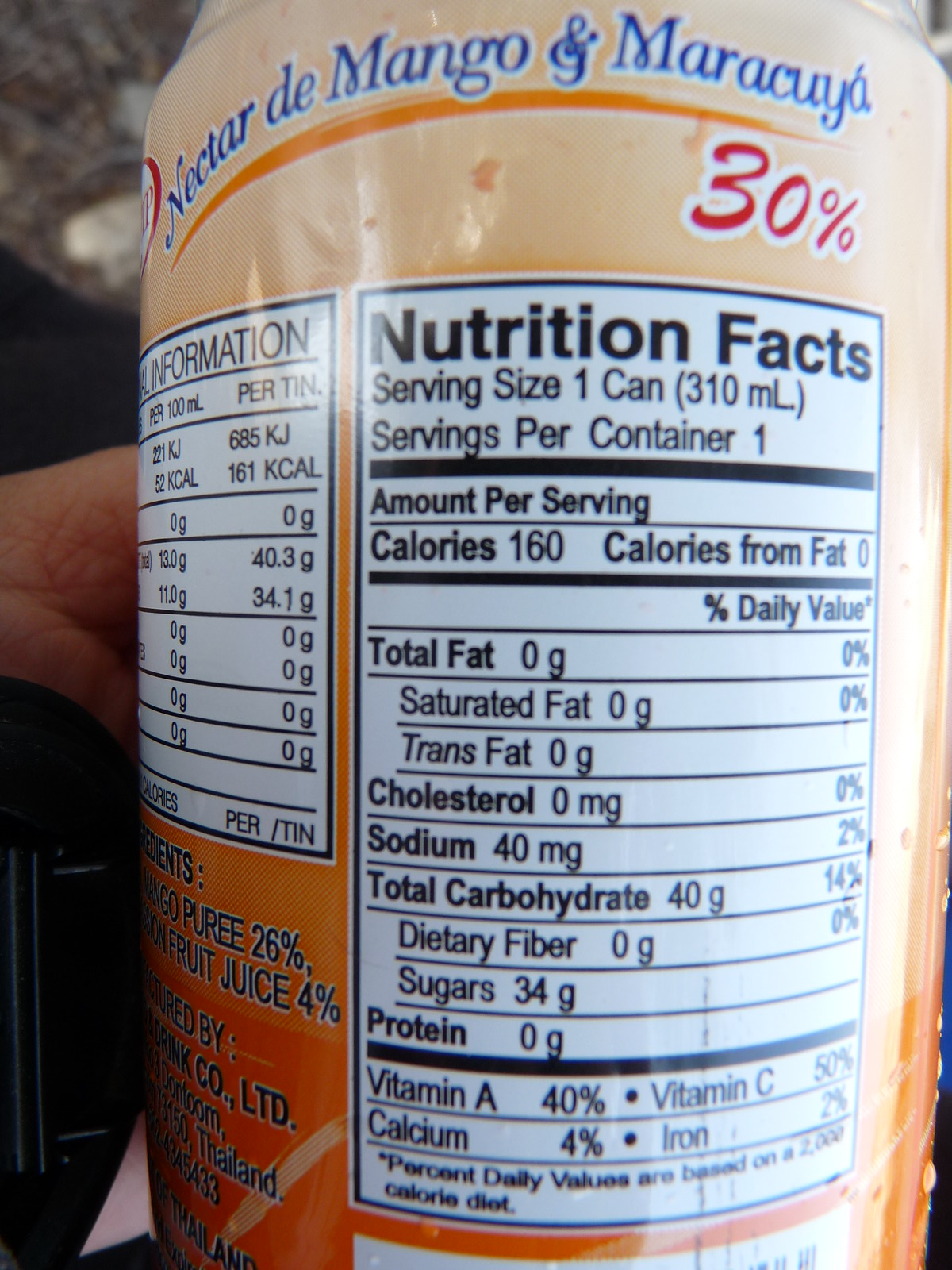The image showcases the side or back of a drink can with a peach-colored exterior. Prominently displayed at the top in blue writing are the words "Nectar Day Mango and Marikea 30%." Below this, the nutritional facts label is clearly visible, printed on a completely white background with black text. The detailed label includes the following information:

- **Serving Size**: 1 can (310 milliliters)
- **Servings Per Container**: 1
- **Calories**: 160
- **Calories from Fat**: 0
- **Total Fat**: 0g (0%)
- **Saturated Fat**: 0g (0%)
- **Trans Fat**: 0g
- **Cholesterol**: 0mg (0%)
- **Sodium**: 40mg (2%)
- **Total Carbohydrates**: 40g (14%)
- **Dietary Fiber**: 0g
- **Sugars**: 34g
- **Protein**: 0g

Additionally, the label provides information on vitamins and minerals:
- **Vitamin A**: 40%
- **Vitamin C**: 50%
- **Calcium**: 4%
- **Iron**: 2%

A note at the bottom clarifies that the percent daily values are based on a 2,000 calorie diet.